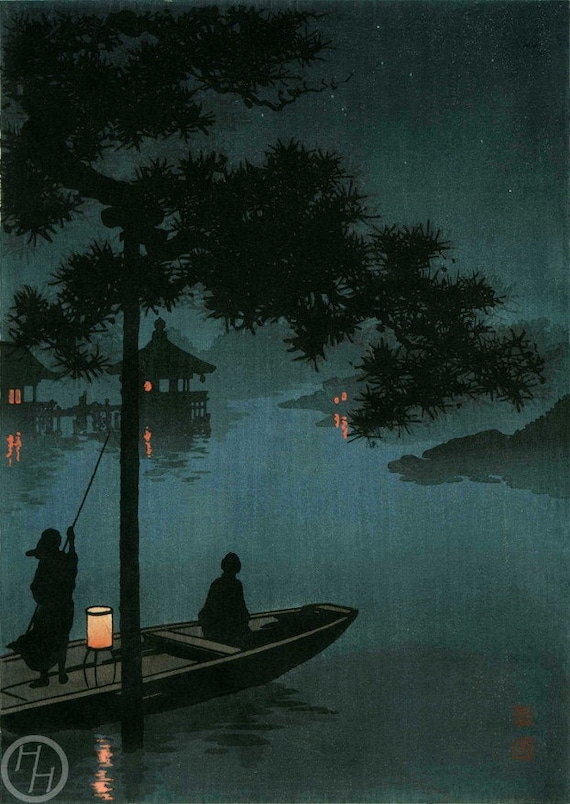The image possesses an illustrative quality reminiscent of book art. In the bottom left corner, there is an artist's signature in an off-white color that gracefully encircles the corner. Dominating the scene are two figures seated in a rowboat. One appears to be a woman standing confidently with longer hair cascading down her back, holding a long pole. Her dress billows behind her in the gentle breeze, adding to the dynamic feel of the scene. A lantern emits an amber glow that softly illuminates the boat and its occupants. The second figure, cloaked in black, is seated towards the front of the boat, their back hunched slightly as they appear deep in thought or contemplation. 

The boat drifts on a serene body of water, surrounded by silhouettes of trees. Rock outcroppings break the smooth surface of the water, adding texture to the background. To the side, two hut-like structures stand on stilts in the water, emitting a warm, soft orange glow that reflects subtly on the water's surface. The entire scene is rendered in a palette of blacks, blues, and whites, creating a tranquil yet mysterious atmosphere. Above, a starry sky stretches out, adding a sense of depth and wonder to the composition.